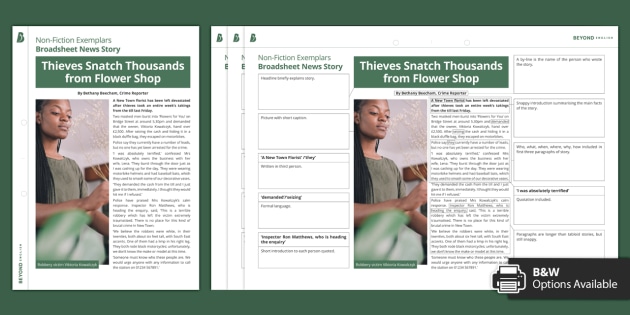The image is a screenshot of what appears to be an educational page likely intended for teachers or individuals in the educational sector. The layout incorporates two main sections. On the left, there's a green header with the title "Nonfiction Exemplars, Broadsheet News Story." Below the header, in larger font and set against a deep green background, the article headline reads "Thieves Snatched Thousands from Flower Shop" accompanied by a picture of an African woman in a gray shirt who looks determined. To the right of this section, the same headline and image are repeated, forming the central part of what resembles a worksheet. Around this repeated article are several rectangular boxes with smaller questions and blank spaces for answers, suggesting that these are areas meant for student responses. The background and the worksheet are primarily white with black text. Notably, on the bottom right of the image, there is an icon of a printer next to a black banner with white text that states, "B&W options available."